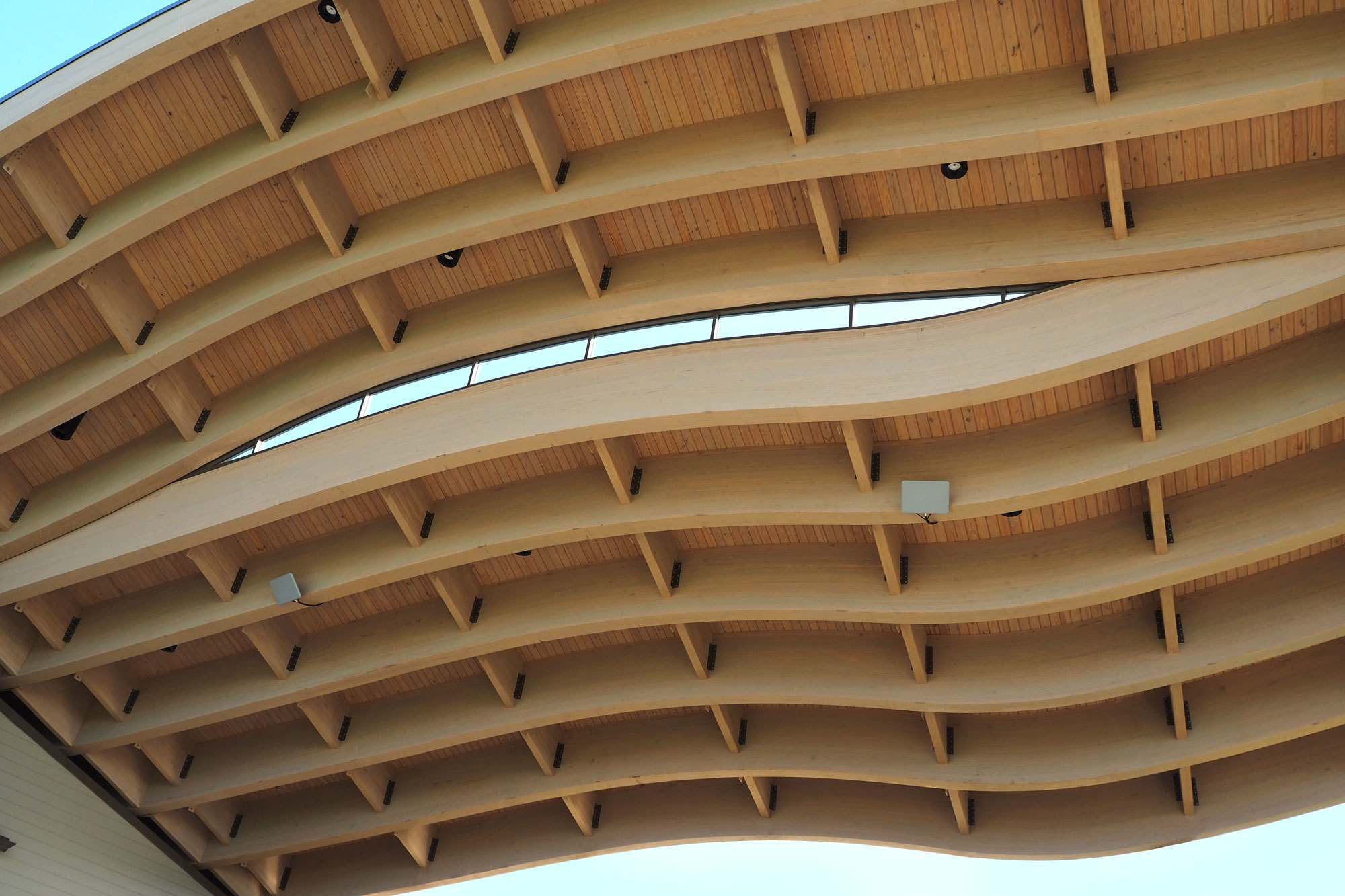The image shows the underside of an outdoor wooden walkway structure, possibly part of an elevated theater or park pathway. The vantage point is from below, looking up at two distinct curving bridges, each with visible guardrails and made of light-colored wooden planks. Large beams run perpendicular to the slats, supporting the structure with a vertical wave pattern. One bridge curves up and then down, while the other goes straight before dipping and rising again. You can see a clear blue sky with a slight green tinge above, and minimal walls or other structures, suggesting it might be an atrium or open space. Lights are visible beneath the bridges, aiding those walking underneath, and portions of white brickwork can be spotted on the left.